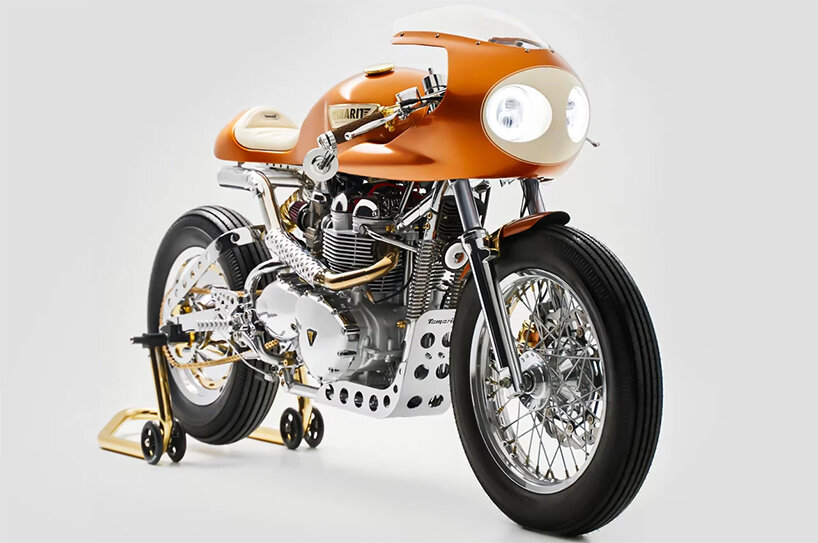The detailed photograph showcases an orange and chrome motorcycle, often referred to as a "crotch rocket" due to its design where the rider leans forward to drive. The motorcycle features an eye-catching orange plastic shell covering areas like the front light housing, gas tank, and seat. The seat itself is cushioned and white. Prominent chrome elements dominate the body, except for the tires. Notably, the motorcycle rests on training wheels, suggesting it's set up for maintenance, allowing the engine to be revved without moving the bike. The machine boasts two large, bright headlights, spaced apart and resembling the eyes of a bee. The background is stark white, indicating that this professional photograph was likely intended for advertisement or magazine use. The bike’s structure is clearly visible with all essential mechanical components exposed between the wheels and under the seat, complemented by a front mudguard and a protective plastic or glass guard.